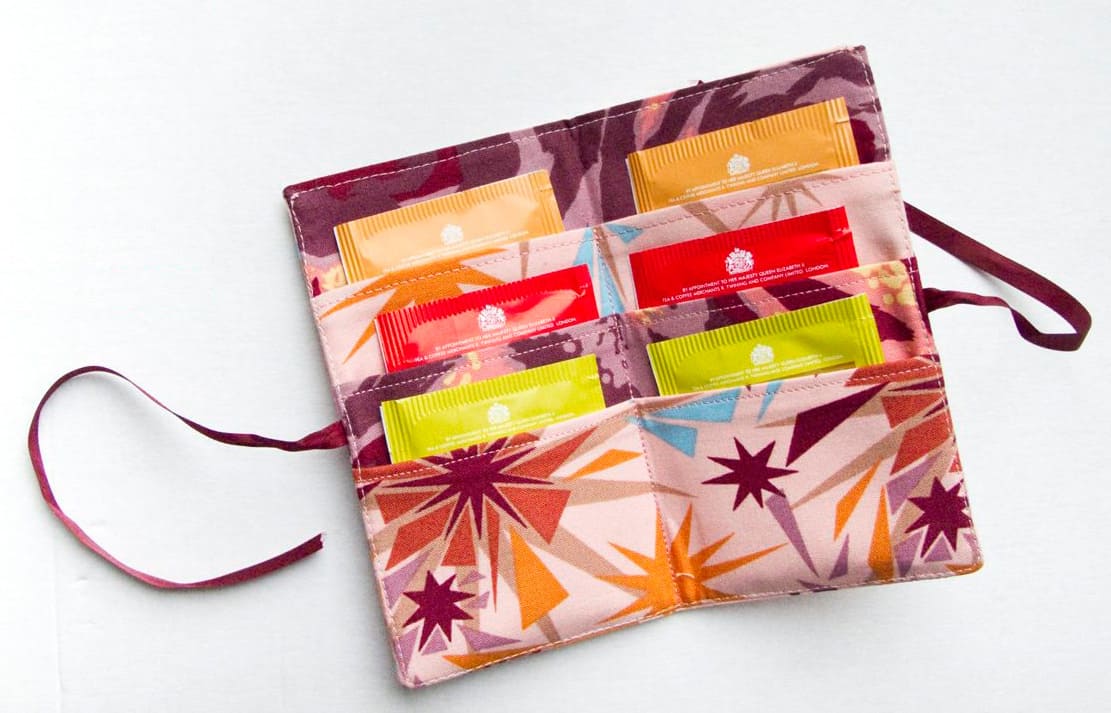This horizontally aligned, rectangular image showcases a textured white background with slight dents on the lower left side. Positioned on the background is a fabric bifold wallet, adorned with a pattern of stars and triangles in burgundy, maroon, orange, yellow, and lavender hues. The wallet features three pocket compartments on each side, enclosed by a burgundy ribbon on both ends to tie it shut. In each of these compartments, packages—resembling tea bags or hand wipes—jut out. The bottom two packages are bright yellow with a white logo, the middle two are red with a white logo, and the top two are orange with a white logo. A small tear strip is visible on each package, indicating an easy-open feature. When the wallet is open, it forms an almost square shape, revealing both its design and the neatly organized contents within.